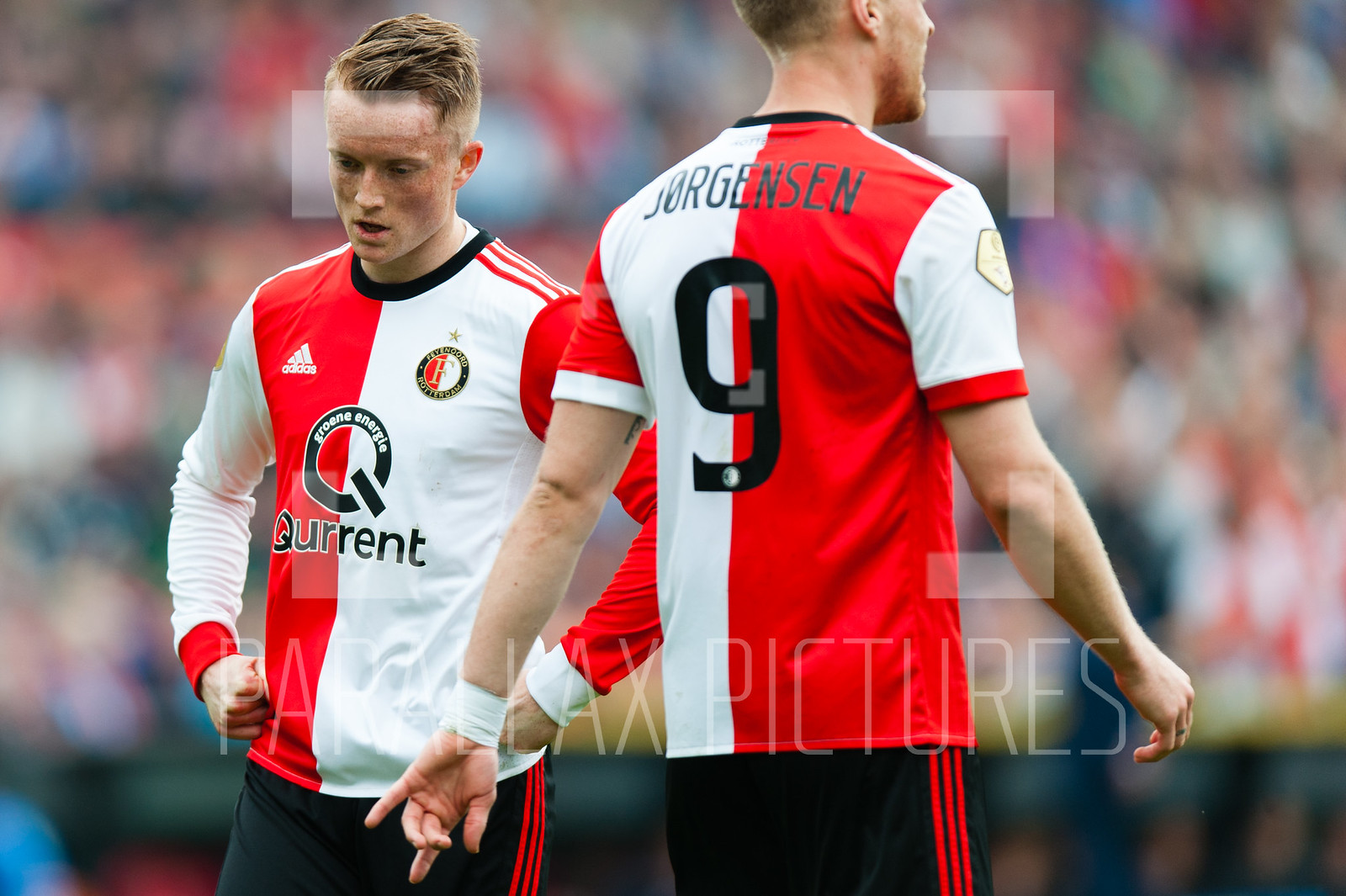The image depicts two young white male soccer players, likely in their 20s or 30s, both with blonde hair, in the midst of a soccer game. They are both wearing identical red, white, and black uniforms with an Adidas logo on the left side of their jerseys. The front of their jerseys feature the logo "Q-U-R-E-N-T" prominently. The player on the left is shown from the front, while the player on the right, with "Jorgensen" and the number nine on the back of his jersey, is seen from behind. In the background, there is a large but blurred crowd. Additionally, there is a watermark from Parallax Pictures in the middle of the image.